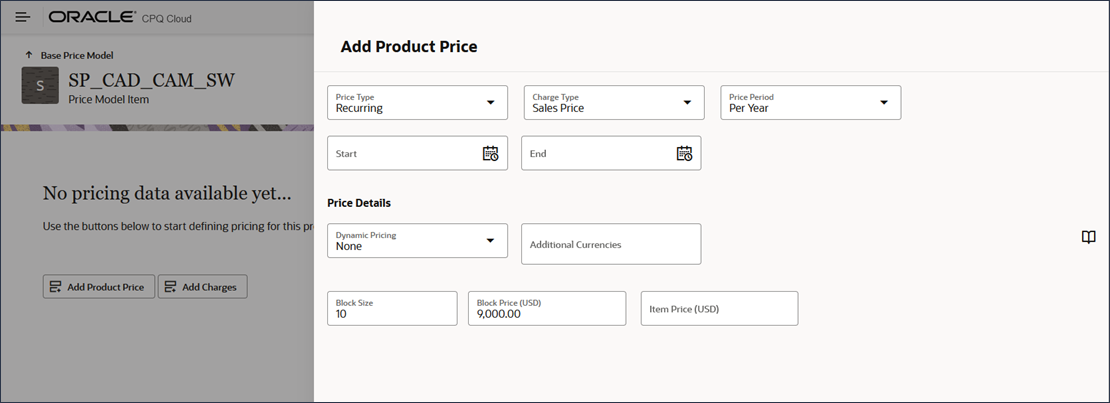**Detailed Descriptive Caption:**

The image showcases a user interface in Oracle’s CPQ Cloud, featuring a comprehensive layout for dynamic pricing models. On the far left corner, three horizontal lines are stacked, symbolizing the Oracle CPQ Cloud menu. Below the three lines, there's a section covered by a semi-transparent gray overlay. This section's top part contains upward arrows labeled "Base Price Model".

Adjacent to the arrows, there is a black square with a white "S" inside, followed by the text: "SP_CAD_CAM_SW Price Model Item". Below this, a multi-colored band separates the previous section from the next, which returns to a white background with the message: "No pricing data available yet. Use the buttons below to start defining prices for this PR..." – however, the text gets cut off mid-sentence.

Under this message are two prominent buttons labeled "Add Product Price" and "Add Charges". On the right side of the interface, another "Add Product Price" button appears. Beneath this, there is a dropdown menu for selecting "Price Type" which currently displays "Reoccurring". Below this is another field labeled "Charge Type" that shows "Sales Price," accompanied by a pull-down menu indicating "Price per Period per Year".

Further down, the interface shows an empty "Start Date" field with a calendar icon nearby, presumably for selecting dates, but no date is specified. The "Price Details" section mentions "Dynamic Pricing" with a drop-down menu set to "None". Below this, an "Additional Currencies" section appears but does not currently display any options.

The "Block Size" field is set to 10, and next to it, the "Block Price" is listed as USD $9,000. Finally, there's an “Item Price” field at the bottom that remains empty.

This detailed layout is designed for users to manage and define various pricing components for products within Oracle CPQ Cloud.